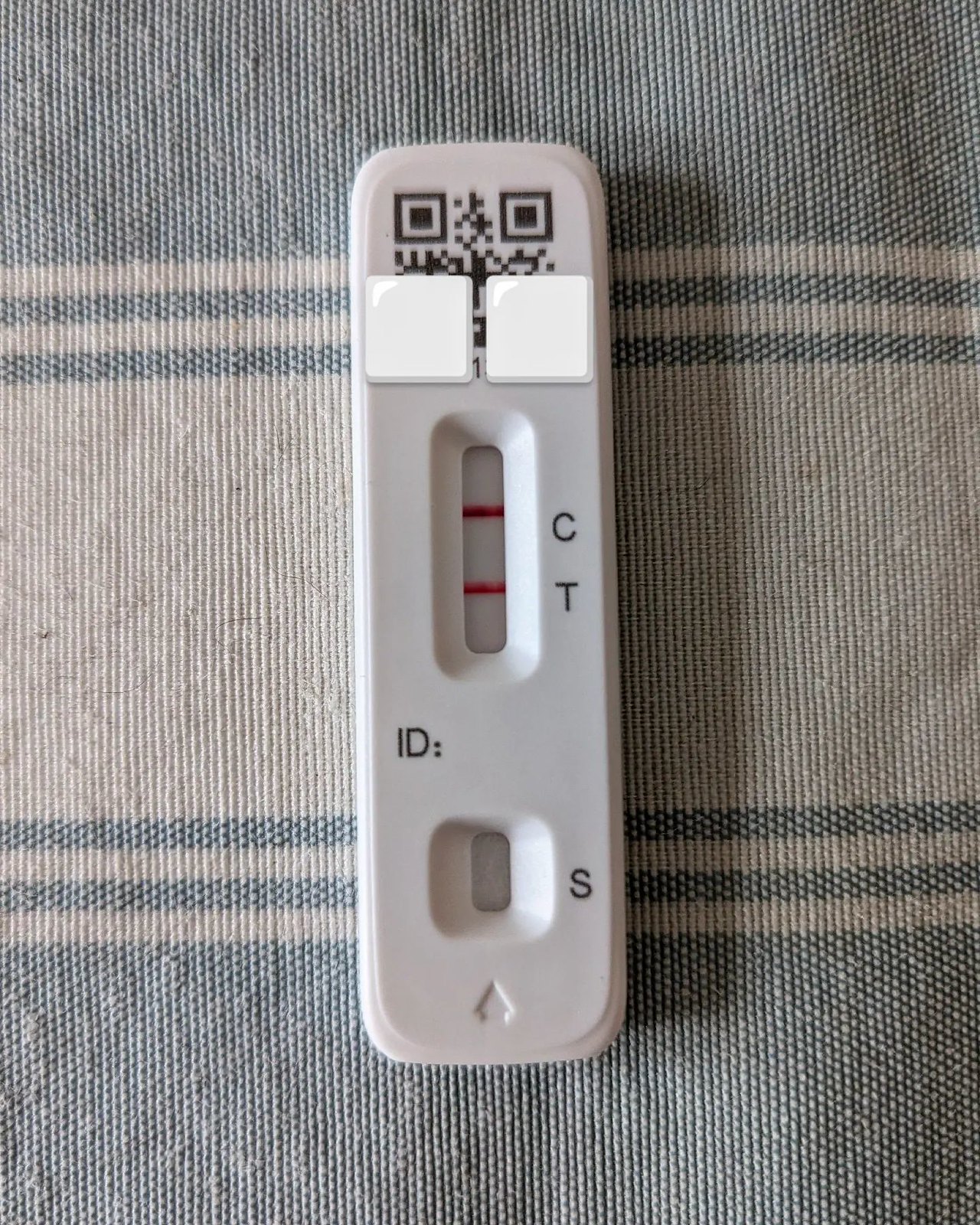This image is a close-up of a white COVID-19 test resting on a patterned dish towel. The towel features a blue border at the bottom, followed by alternating skinny horizontal stripes: white, blue, white, blue, and a solid white center, and the same pattern reversed on the opposite side. 

The COVID-19 test itself is slightly wider and thicker than a typical pregnancy test. At the bottom, it has an arrow pointing upwards. There is a small window with the letter 'S' in black next to it. Above this, on the left, the label 'ID:' is printed. Further up, there is a larger window displaying the test results, which is approximately three times the size of the bottom window. Inside this larger window, two solid red lines are visible, with a 'C' next to the top line and a 'T' next to the bottom line. 

Above the results window, a QR code is partially visible; two white square stickers obscure the bottom part of the QR code, leaving only the top part visible. Based on the structural features and context, the test appears to be a COVID-19 rapid antigen test rather than a pregnancy test.